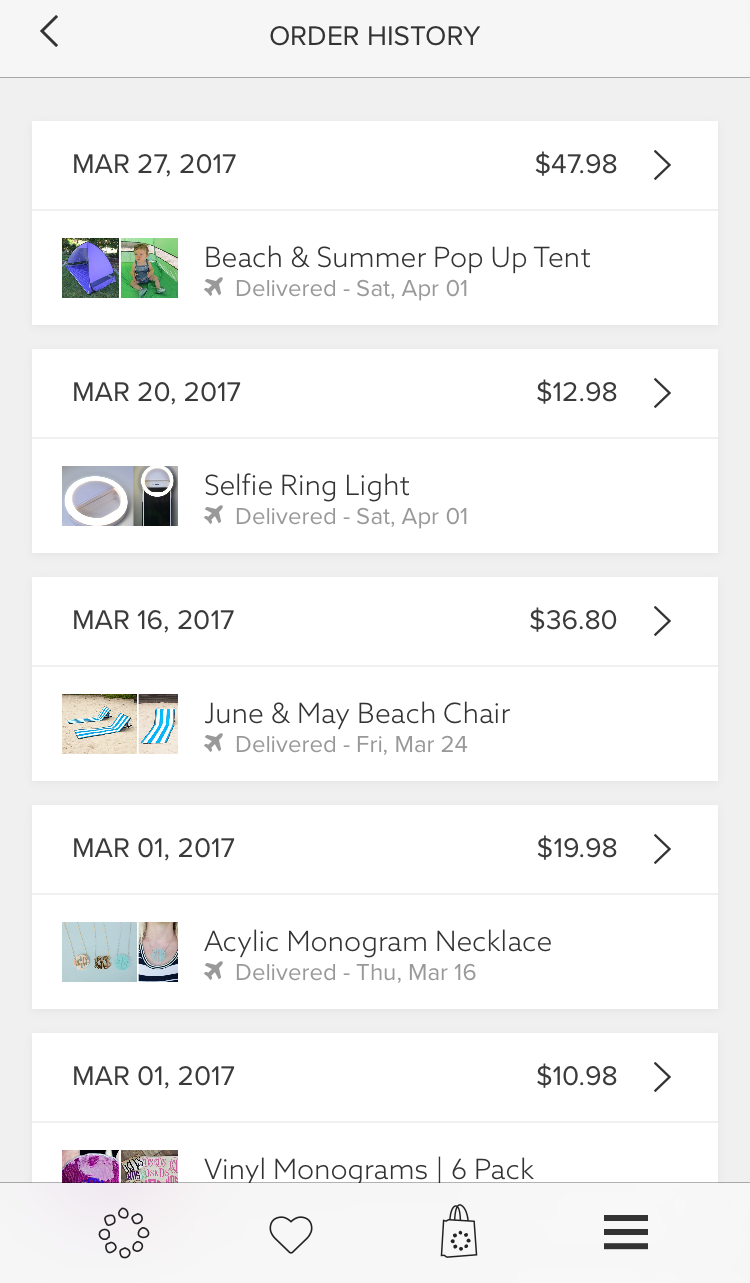Screenshot of Mobile Order History

This image is a screenshot captured from a mobile device, showcasing an app's order history page. The layout is vertically rectangular, characteristic of smartphone screens. At the top of the page, the title "Order History" is prominently displayed, accompanied by a left-arrow icon on the left edge, likely for navigation.

Below the header, the screen lists five distinct order entries in separate white boxes. Each entry includes the order date, the purchase details, delivery status, and small thumbnail images representing the items.

1. **Order 1:**  
   - **Date:** March 27, 2017
   - **Item:** Beach and Summer Pop-Up Tent
   - **Price:** $47.98
   - **Delivery Date:** Delivered on Saturday, April 1, 2017
   - **Thumbnails:** Two small images of the pop-up tent
   - **Additional Icon:** Airplane symbol next to the delivery status

2. **Order 2:**  
   - **Date:** March 20, 2017
   - **Item:** Selfie Ring Light
   - **Price:** $12.98
   - **Delivery Date:** Delivered on Saturday, April 1, 2017
   - **Thumbnails:** Image of the selfie ring light
   - **Additional Icon:** Airplane symbol next to the delivery status

3. **Order 3:**  
   - **Date:** March 16, 2017
   - **Item:** June and May Beach Chair
   - **Price:** $36.80
   - **Delivery Date:** Delivered on Friday, March 24, 2017
   - **Thumbnails:** Image of the beach chair
   - **Additional Icon:** Airplane symbol next to the delivery status

4. **Order 4:**  
   - **Date:** March 1, 2017
   - **Item:** Acrylic Monogram Necklace
   - **Price:** $19.98
   - **Delivery Date:** Delivered on Thursday, March 16, 2017
   - **Thumbnails:** Image of the necklace
   - **Additional Icon:** Airplane symbol next to the delivery status

5. **Order 5:**  
   - **Date:** March 1, 2017
   - **Item:** Vinyl Monogram Six-Pack
   - **Price:** $10.98
   - **Delivery Date:** Delivered on March 1, 2017
   - **Thumbnails:** Image of the vinyl monogram
   - **Additional Icon:** Airplane symbol next to the delivery status